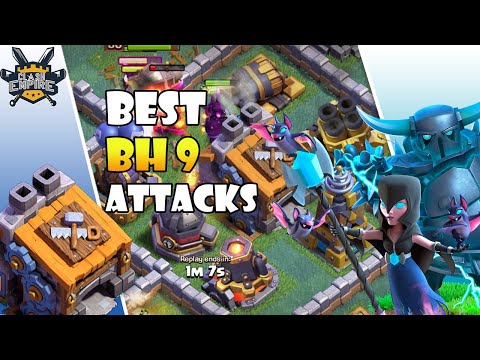The image depicts a digital screenshot from a Clash of Clans themed video game, designed to be a clickable screen similar to a YouTube thumbnail. This image features a prominent black bar at the top and bottom. In the top left corner, there is a yellow castle-like icon with the gray text "Clash Empire" overlaid. Behind this text are two crossed swords, visible by their hilts at the bottom left and bottom right, and their tips at the top left and top right. 

Dominating the center of the image are several structures encircled by a gray wall, indicating a base or home base in the game. Centrally positioned is bold text that reads "Best" in white, followed by "BH9" in yellow, and "Attacks" in white. Under this, slightly smaller text displays "1M7S" in white, and even smaller above it, "Replay Enzin" can be seen, though it is quite faint.

To the right are two notable cartoon-like characters: a knight clad in teal armor with large horns on his helmet, and a hooded figure resembling an executioner wielding a large ax. The entire scene is vividly colorful with shades of light blue, blue, black, orange, yellow, green, light green, pink, and gray. The various elements and characters appear to be randomly distributed, contributing to a dynamic, animated aesthetic reflective of a futuristic digital creation.